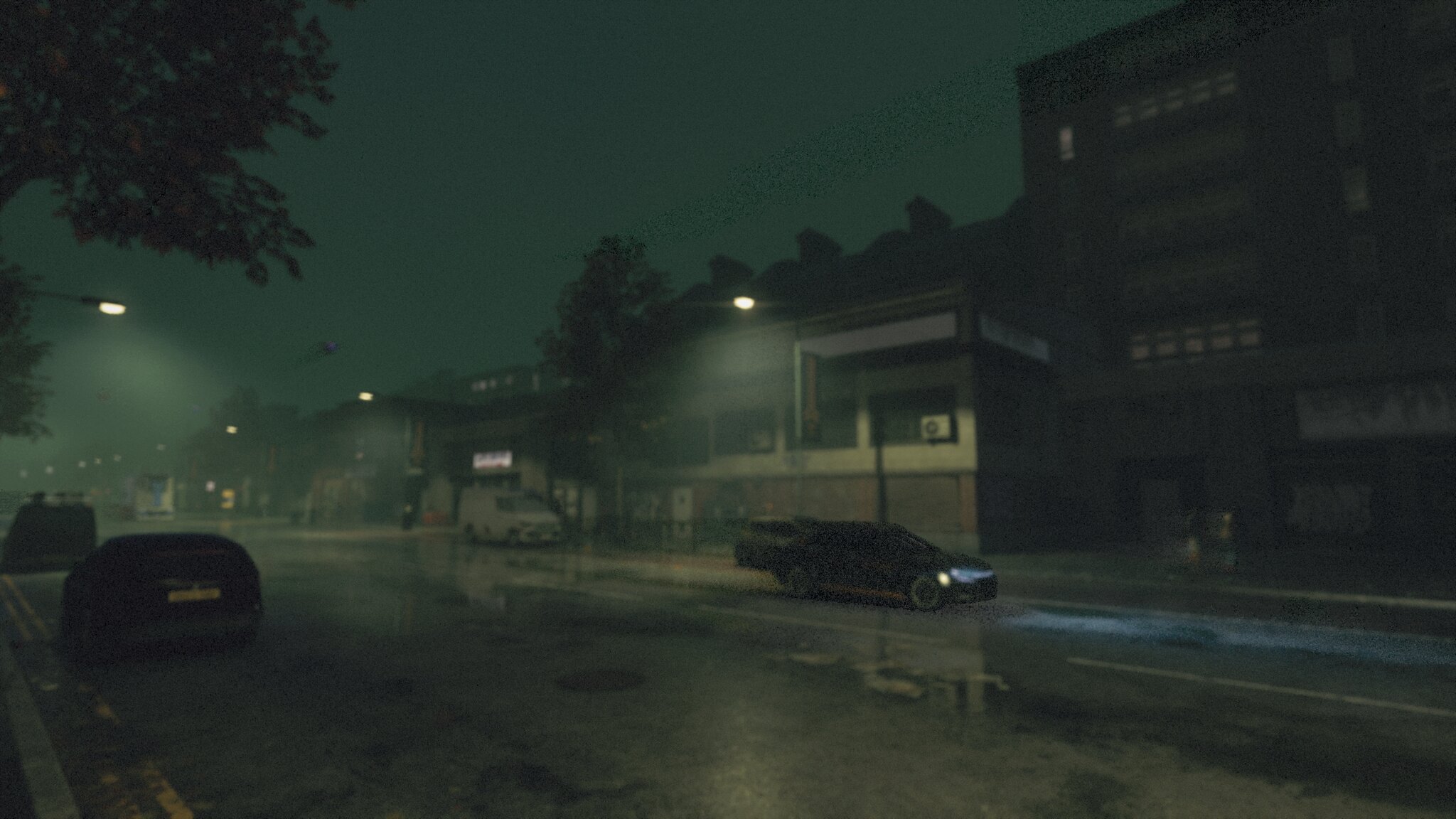The image depicts a low-resolution, grainy nighttime scene most likely from a video game due to several unnatural reflections and atmospheric effects. The rectangular image shows a wet, dirty road lined with parked cars and illuminated by several streetlights, resulting in scattered reflections and a hazy appearance. The scene is potentially set in the UK, inferred from the cars parked on the left side and their positioning on the road. On the near side of the street, multiple vehicles, including a dark-colored car with its headlights on, are visible along with some trees positioned in the top left corner. Across the street, there's a four or five-story brick building, possibly an apartment, library, or hospital, accompanied by several low-level buildings. Additionally, there is a white van parked on the far side with a sign above it. The sky above is a blend of dark black and hints of dark green or purple.